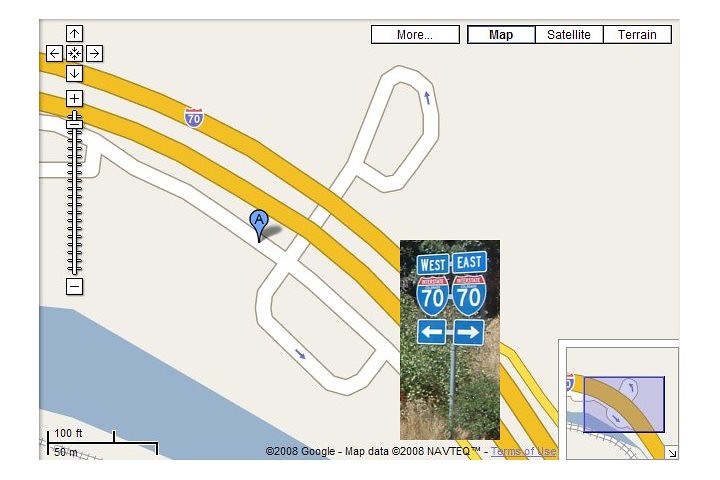This image is a rendered map, likely from Google Maps around 2008, as noted by the copyright markings that read "© 2008 Google, Map Data © 2008 Navteq." The map shows a section of Interstate 70 (I-70), marked prominently in yellow as it runs east-west. There's a marker labeled 'A' situated between the interstate and a nearby river. The map interface includes buttons at the top labeled "Map," "Satellite," and "Terrain," and there is a scale indicator at the bottom left showing distances like 100 feet and 50 meters. Additionally, a small inset map appears in the bottom right corner. Street signs indicating "West" and "East" for I-70 are also visible. Some looping roads are present near the interstate, depicted in white. The image includes navigation tools like zoom buttons, further emphasizing its digital and interactive nature.